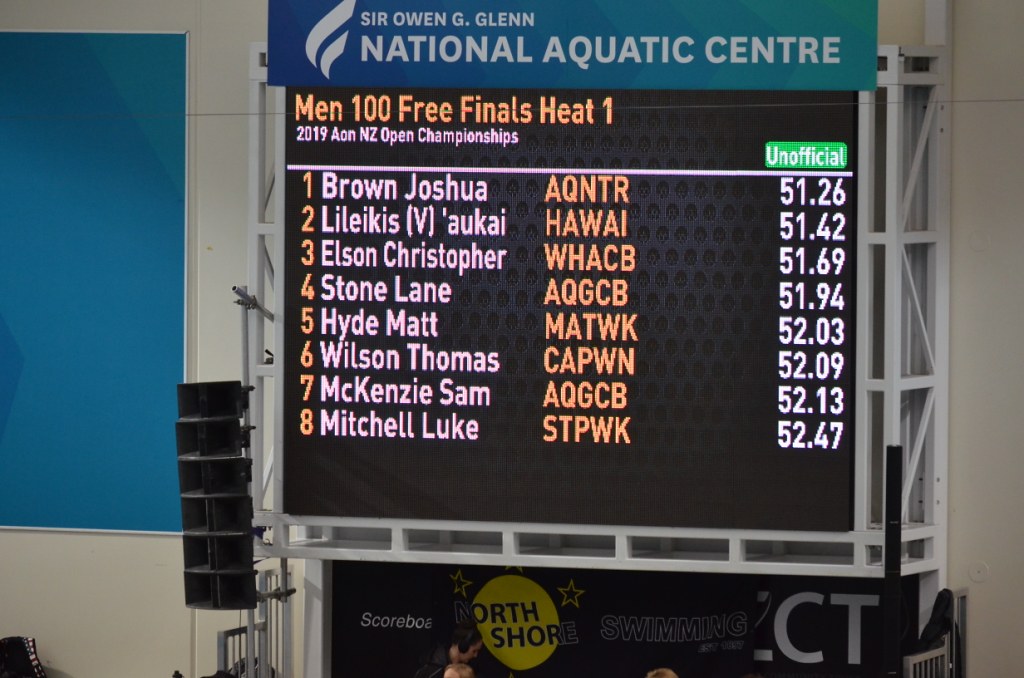The photograph captures an indoor scene, specifically the scoreboard at the Sir Owen G. Glenn National Aquatic Center, evidenced by the artificial lighting. At the top of the scoreboard, a rough blue gradient banner transitions from darker to lighter blue, featuring the National Aquatic Center's name in white text. Below, in green digital text, the scoreboard reads "Men 100 Free Finals Heat 1" and in white text, "2019 AON New Zealand Open Championships." The list displays competitors' names and their unofficial times.

1. Brown Joshua - 51.26
2. Lyle Likas - 51.42
3. Aokai - 51.42
4. Elson Christopher - 51.69
5. Stone Lane - 51.94
6. Hyde Matt - 52.03
7. Wilson Thomas - 52.09
8. Mackenzie Sam - 52.13
9. Mitchell Luke - 52.47